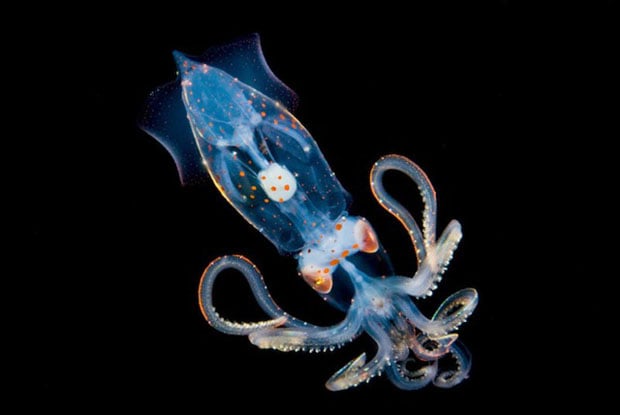The image showcases a large, vibrant blue sea squid set against a completely black background, which highlights its bioluminescent glow. The squid's body is elongated and cylindrical, widening at the top, with a transparent quality that reveals some of its internal organs. Prominent orange eyes flank each side of its head, and a puckered mouth is visible at the front. Its tentacles, symmetrically arrayed, are adorned with numerous white dots and small orange speckles, adding to the fascinating texture of its form. Positioned diagonally across the frame, the creature exudes an ethereal, otherworldly beauty.